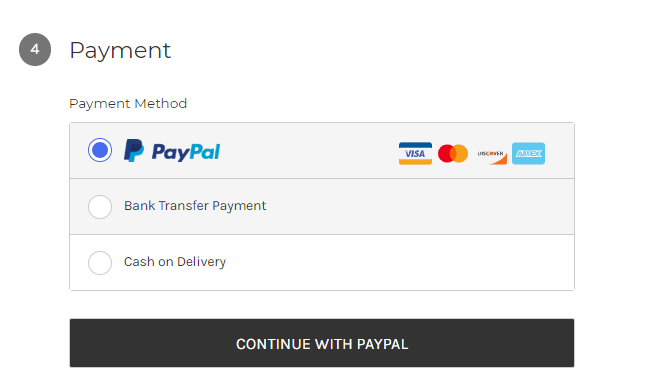The image is a cropped screenshot of a payment screen, focusing solely on the payment box section. At the top left, there's a black bubble with the number "4" in white text. To the right of this bubble, the word "Payment" is prominently displayed in large black letters. Directly below "Payment," spaced slightly further down, are the words "Payment Method" in smaller, gray letters.

Below "Payment Method," a box presents three payment options:

1. **PayPal** - This option is highlighted and selected. To its right, there is an indication that PayPal supports Visa, MasterCard, Discover, and Amex.
2. **Bank Transfer Payment** - Listed under PayPal and contained within a gray section.
3. **Cash on Delivery** - Positioned below Bank Transfer Payment and placed on a white background.

At the very bottom of the section, there is a large, black vertical rectangle. Centered within this rectangle, in white capitalized letters, it says, "CONTINUE WITH PAYPAL."

The image is devoid of any additional graphics or background elements, giving it a distinct appearance as if it's part of a website's interface, but it lacks any visible edges around the payment box.